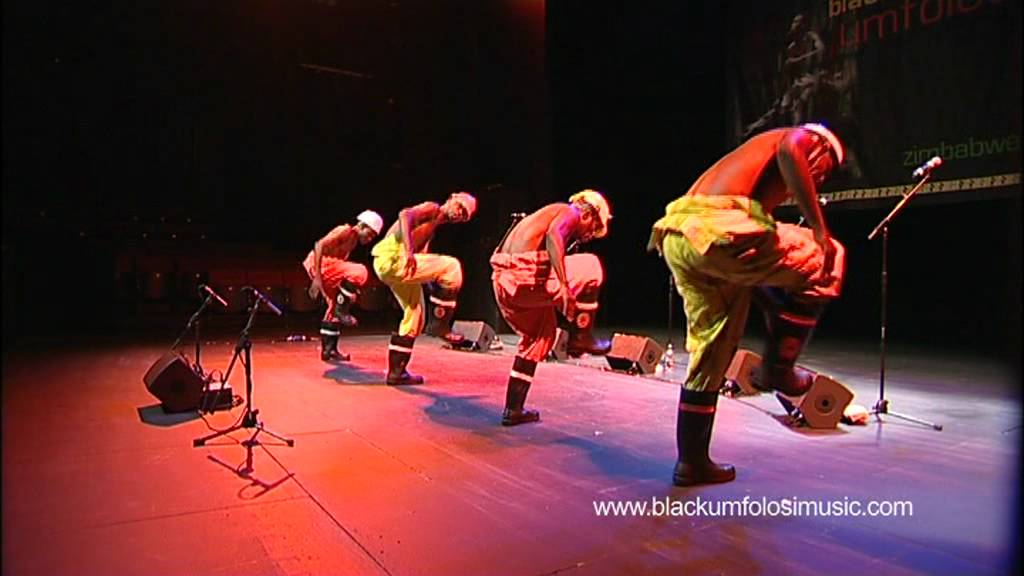The image captures an oblique view of four bare-chested male performers on a stage, each donned in colored construction helmets and yellow overalls that are pulled down to their waists, revealing black rubber boots with white stripes across the calves. The men, lined up and dancing in sync, are all bent over with one leg raised, poised as if about to stomp. Surrounding them are multiple microphones and speaker boxes, with two microphones positioned in front and another set behind them. The stage is illuminated by a light blue light from the front and a red light from the back, creating a contrast against the dark background. The scene exudes a construction or firefighter theme with a hint of a male stripper motif, as suggested by the stripped-down attire and overall setup. The text "www.blackumphalosemusic.com" is visible within the image.